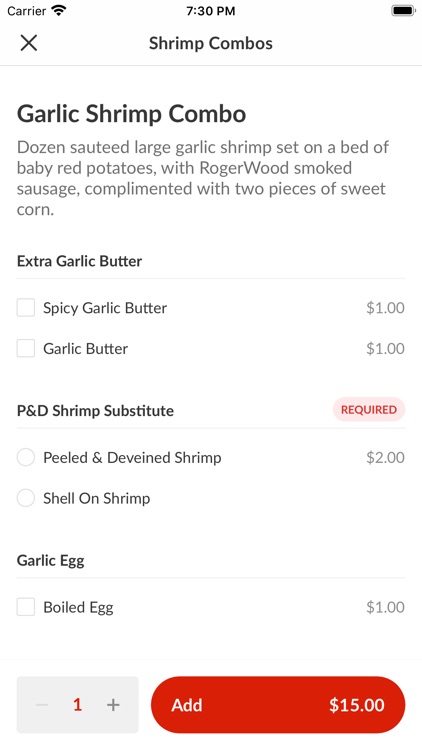A screenshot of a tablet display showcasing an online food ordering app. The screen displays various menu options, Wi-Fi connectivity, and the current time at 7:30 PM with a full battery indicator. There is an "X" under the carrier signal on the left. The central part of the screen features a listing for a "Garlic Shrimp Combo," which includes a dozen sautéed large shrimp set on a bed of baby red potatoes with Roger Wood smoked sausage, complemented by two pieces of sweet corn. 

Additional options include extra garlic butter with a line item showing:
- A check box for "Spicy Garlic Butter" at $1 (unchecked)
- A check box for "Garlic Butter" at $1 (unchecked)

Below this, the display shows an option for "P&D shrimp substitute" with a pink button that says "required." 

Next is an option for “Peeled and Deveined Shrimp" with a $2 surcharge and an unchecked circle.

Following this, there is a "Garlic Egg" option underlined, with a check box for adding a boiled egg at $1. There is a field to enter the quantity, showing '1' in red text. 

At the bottom, a red button indicates "Add $15" for the total order.